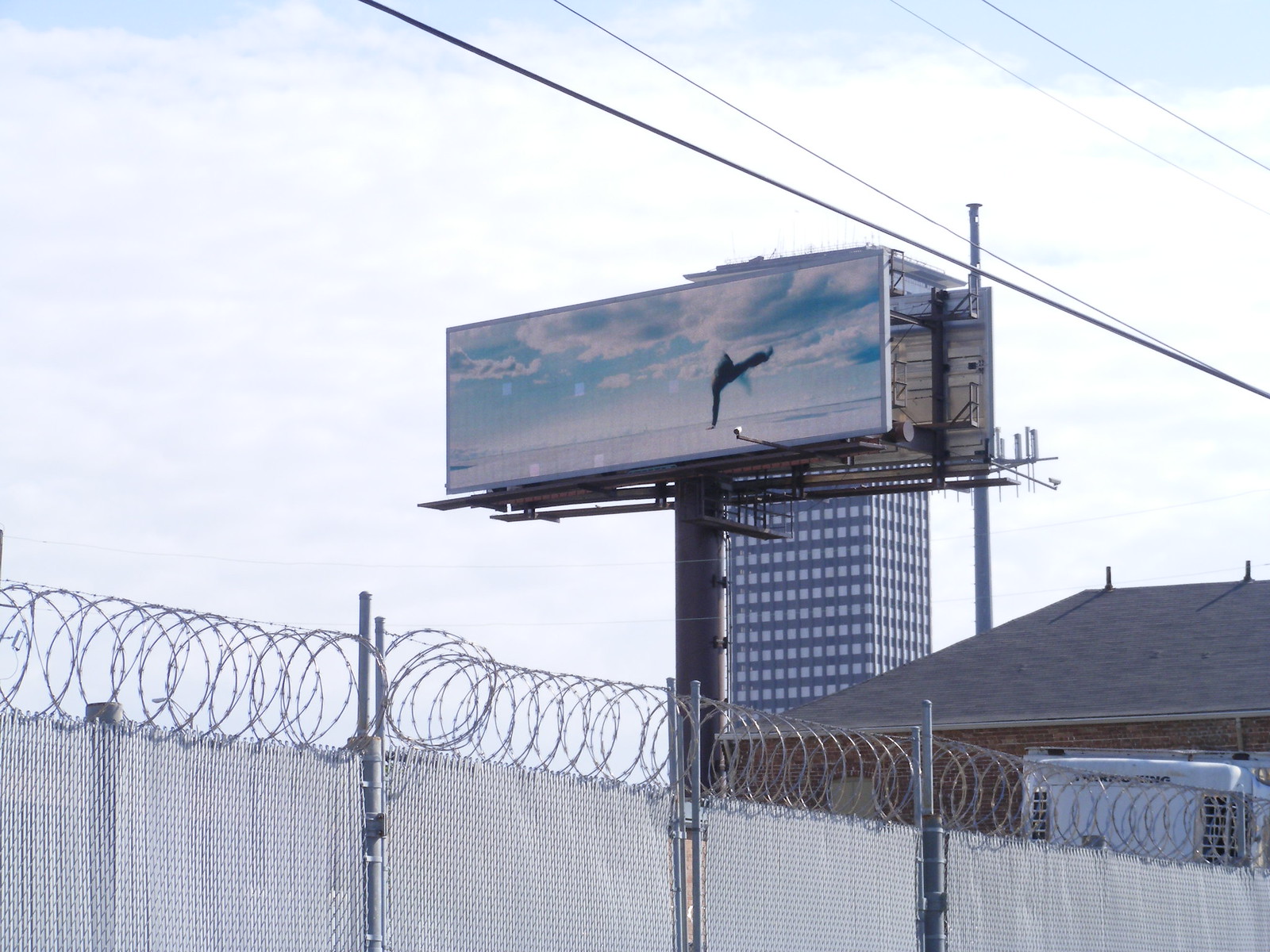Under a brilliant blue sky dotted with fluffy white clouds, a scene is framed by a chain-link fence topped with barbed wire. The fence is supported by metallic poles spaced evenly along its length. Beyond the fence, there is a brown wall extending horizontally, partially obscured by a gray rooftop. To the left, a white truck is parked, while on the right, another vehicle can be faintly made out. Dominating the background is an imposing office building, remarkably tall and lined with numerous windows. Adjacent to this building, a large blue billboard catches the eye, set against the sky and featuring some indistinct black markings. Further behind, yet another billboard is visible, creating a layered urban landscape.